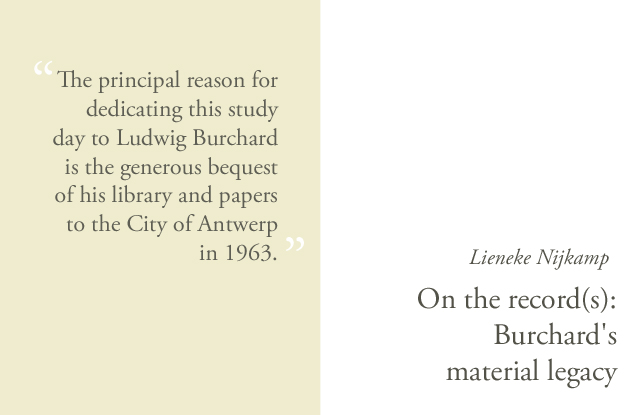The image depicts a two-part layout reminiscent of an educational slide or a book page. On the left side, there is a tan box with black text, surrounded by white quotation marks. The text reads: "The principal reason for dedicating this study day to Ludwig Burchard is the generous bequest of his library and papers to the city of Antwerp in 1963." On the right side, positioned at the bottom right, there is additional black text on a white background stating: "Leineke Nijkamp, on the record, Burchard's material legacy." The color scheme includes tan, black, white, and brown, with no other elements or objects present in the image.